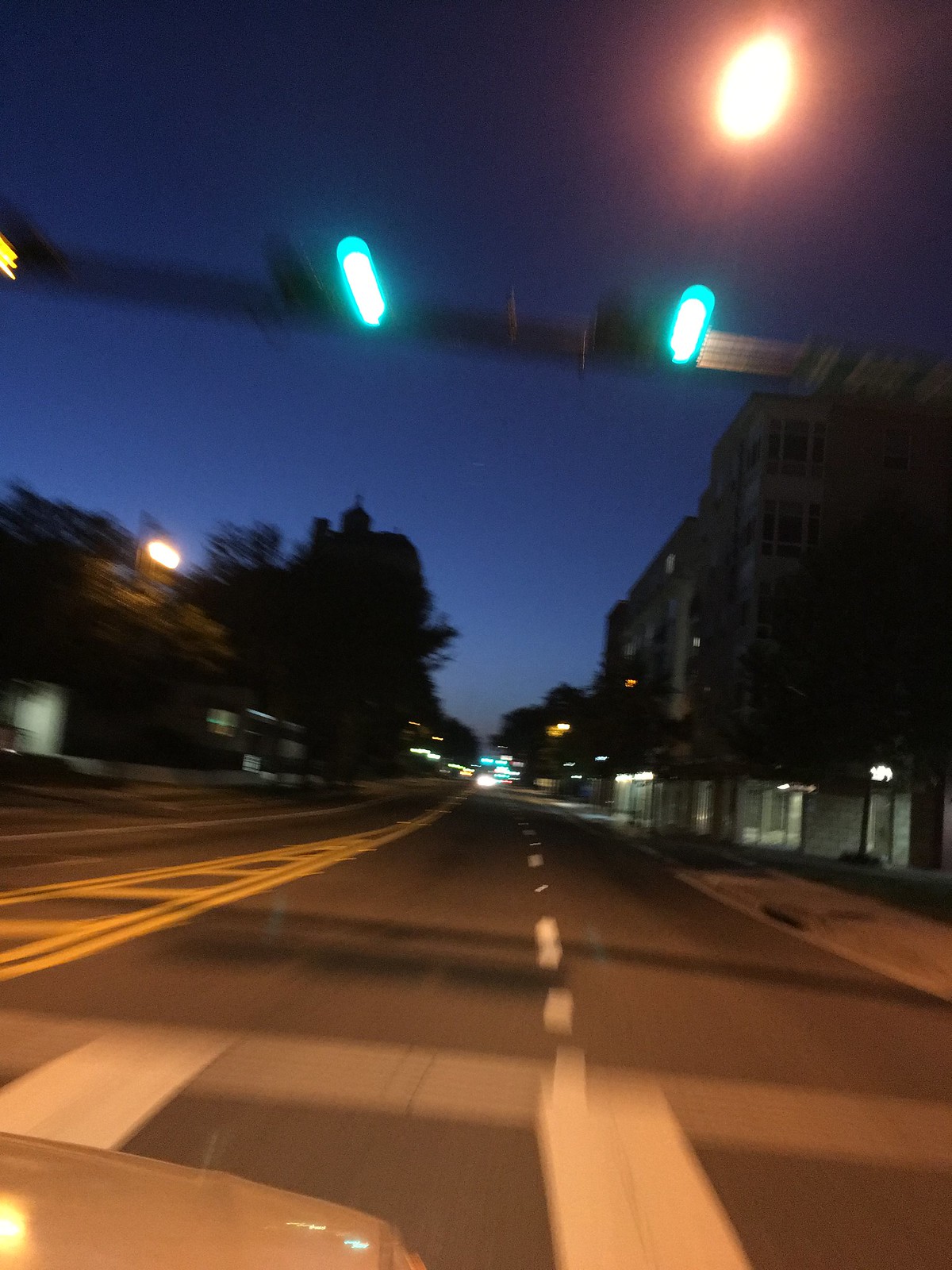A vibrant nighttime color photograph captures a slightly blurred view through the windshield of a vehicle, likely from the driver's perspective. In the bottom left corner, the curved, reflective surface of a rear-view mirror is visible, tinted with light reflections. The focus is on a dimly lit road ahead, featuring a white center line and intersecting road markings, with additional yellow lines visible to the left. Dominating the upper portion of the frame, a deep blue sky fades to darker tones towards the edges, with a subtle, lighter blue gradient in the middle. Overhead, bars likely supporting traffic lights span the road; two traffic lights can be seen glowing green but appear blurry and distorted. In the upper right, a larger round streetlight emits a warm, orangey hue, contrasting with the cooler tones of the scene. Silhouettes of trees line the left side of the road, while distant car lights and faint outlines of tall buildings with illuminated lower sections populate the right side, adding depth and urban ambiance to the scene.